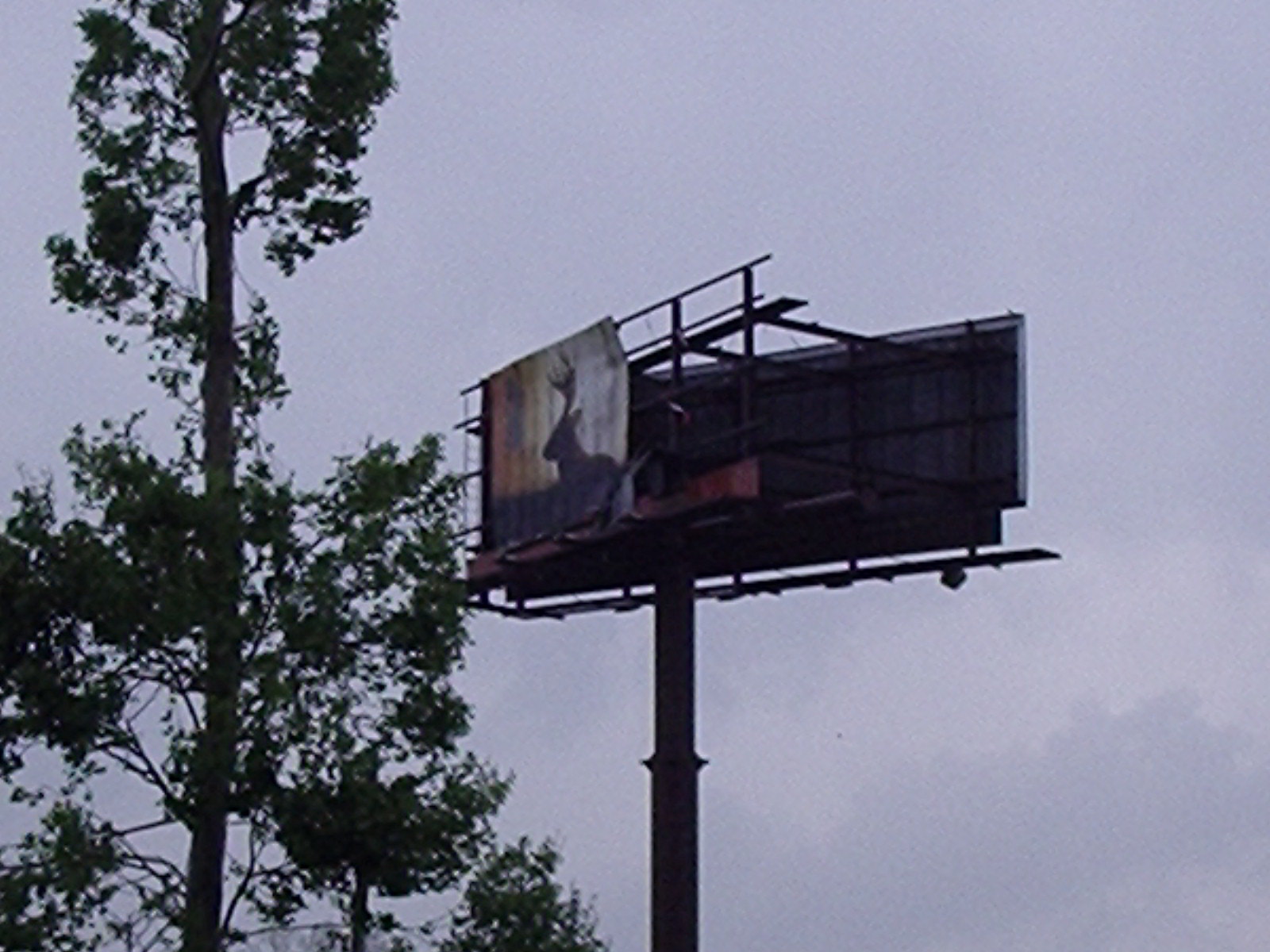In this atmospheric photograph, a dilapidated advertising billboard stands prominently against a moody, grey, cloud-filled sky. The billboard, positioned centrally, is mounted on a tall, stark black pole, further emphasized by the shadowy lighting. The left side of the frame features a large, somewhat shadowed pine tree, with a few visible branches and leaves. 

On the upper left corner of the billboard, an image of a deer with large antlers remains visible, though the picture is heavily rusted, torn, and worn, suggesting years of neglect. The right side of the billboard is missing, exposing metal braces and giving the advertisement a broken, abandoned appearance. A red strip is noticeable at the bottom of the remaining image, possibly part of the frame, painted on what seems to be corrugated iron. All these elements together create a stark and haunting visual, emphasizing decay and abandonment.